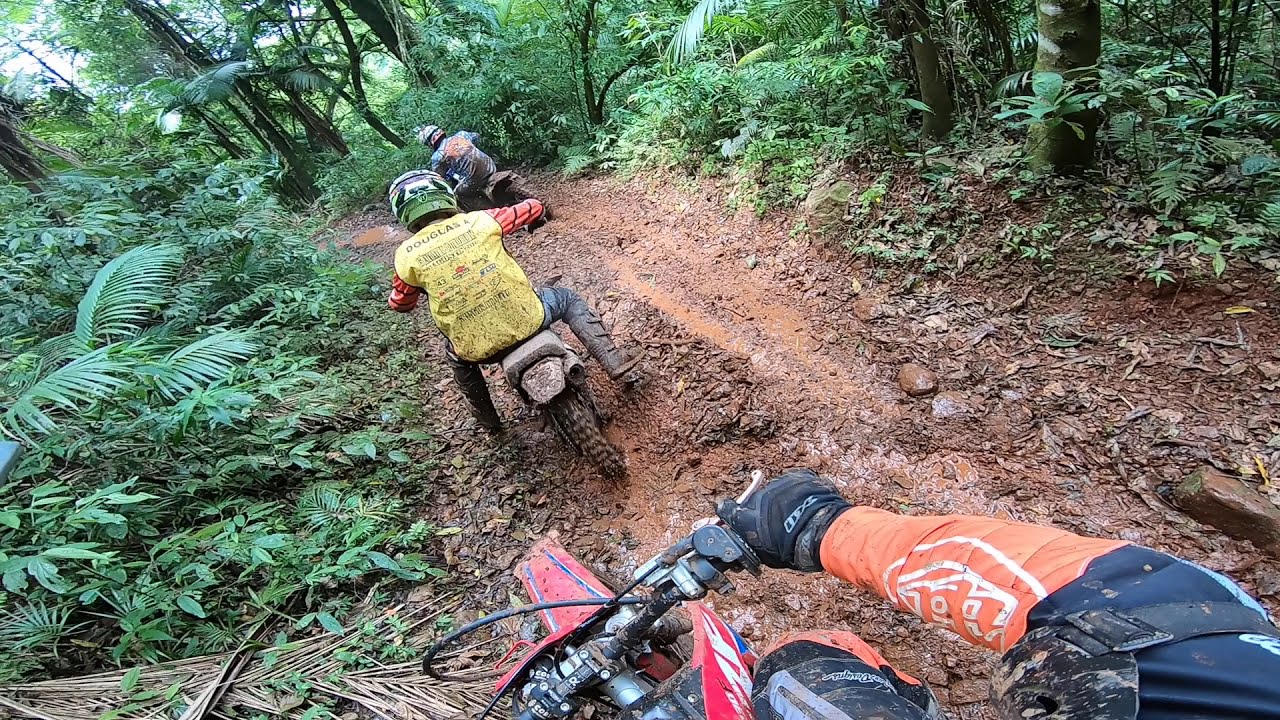In this dynamic daytime photograph, a group of motocross riders are navigating a rugged, muddy trail through a dense, tropical forest. The image is captured from a first-person perspective, likely by a camera mounted on the helmet of the photographer, whose arm clad in an orange-sleeved outfit and black gloves is visible gripping the black handlebars of a red-accented dirt bike. The trail, coated in a brownish-orange, muddy soil, winds to the left, surrounded by lush greenery composed of ferns, palm fronds, and other tropical vegetation. 

Ahead of the photographer, two riders are visible. The nearest one is on a gray motorcycle, donned in a yellow shirt with red sleeves and a green helmet. Further up, another rider can be seen wearing a blue shirt with a matching blue helmet. Both riders are thoroughly splattered with mud, indicative of an intense and challenging ride. The ambient lushness and foliage, combined with the muddy terrain, clearly emphasize the tropical climate and the demanding nature of their excursion.